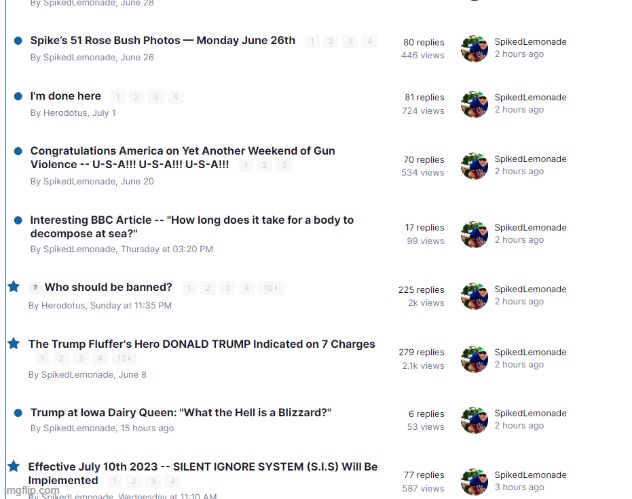Here is a polished and detailed caption for the provided image:

---

**Listing of Articles by Spiked Lemonade**

The image displays a list of articles authored by Spiked Lemonade, set against a white background with black text. Key details of the articles are organized in a bullet-point format, with a vertical blue line running along the far left side of the image. 

At the top left corner, the text "By Spiked Lemonade, June 28th" is prominently displayed in black. Below that is the title "Spikes 51 Rosebush Photos" also by Spiked Lemonade, dated June 26th, with 80 replies and 446 views.

Adjacent to these texts, on the right, there is a circular image of a Caucasian man wearing sunglasses and a blue t-shirt. Next to the image is the name "Spiked Lemonade" with a timestamp of "2 hours ago." 

Proceeding downward:

- "I’m done here" by Herodotus, dated July 1st, shows 81 replies and 124 views, followed by the same circular picture and "Spiked Lemonade, 2 hours ago."
  
- "Congratulations, America, on Yet Another Weekend of Gun Violence — U.S.A!!! U.S.A!!! U.S.A!!!" has 70 replies and 534 views, accompanied by the same picture and "Spiked Lemonade, 2 hours ago."

- "Interesting BBC Article: How Long Does It Take for a Body to Decompose at Sea," by Spiked Lemonade, marked Thursday at 3:20 PM, has 17 replies and 99 views, followed by the picture and "Spiked Lemonade, 2 hours ago."

Next in the listing, there are entries marked with stars instead of bullet points:

- "Who Should Be Banned?" by Herodotus, dated Sunday at 11:35 PM, has 255 replies and 2k views, followed by the picture and "Spiked Lemonade, 2 hours ago."

- "The Trump Fluffer's Hero, Donald Trump, Indicated on 7 Charges," by Spiked Lemonade, dated June 8th, has 279 replies and 2.1k views, followed by the picture and "Spiked Lemonade, 2 hours ago."

Following these starred entries:

- "Trump at Iowa Dairy Queen: What the Hell is a Blizzard?" by Spiked Lemonade, 15 hours ago, with 6 replies and 53 views, accompanied by the picture and "Spiked Lemonade, 2 hours ago."

- "As of July 10th, 2023, Silent Ignore System (SIS) Will Be Implemented," by Spiked Lemonade, stated Wednesday at 11:10 AM, has 77 replies and 587 views, followed by the picture and "Spiked Lemonade, 3 hours ago."

---

This image effectively categorizes and presents the recent articles by Spiked Lemonade, accurately detailing their authorship, dates, interactions, and visuals associated.